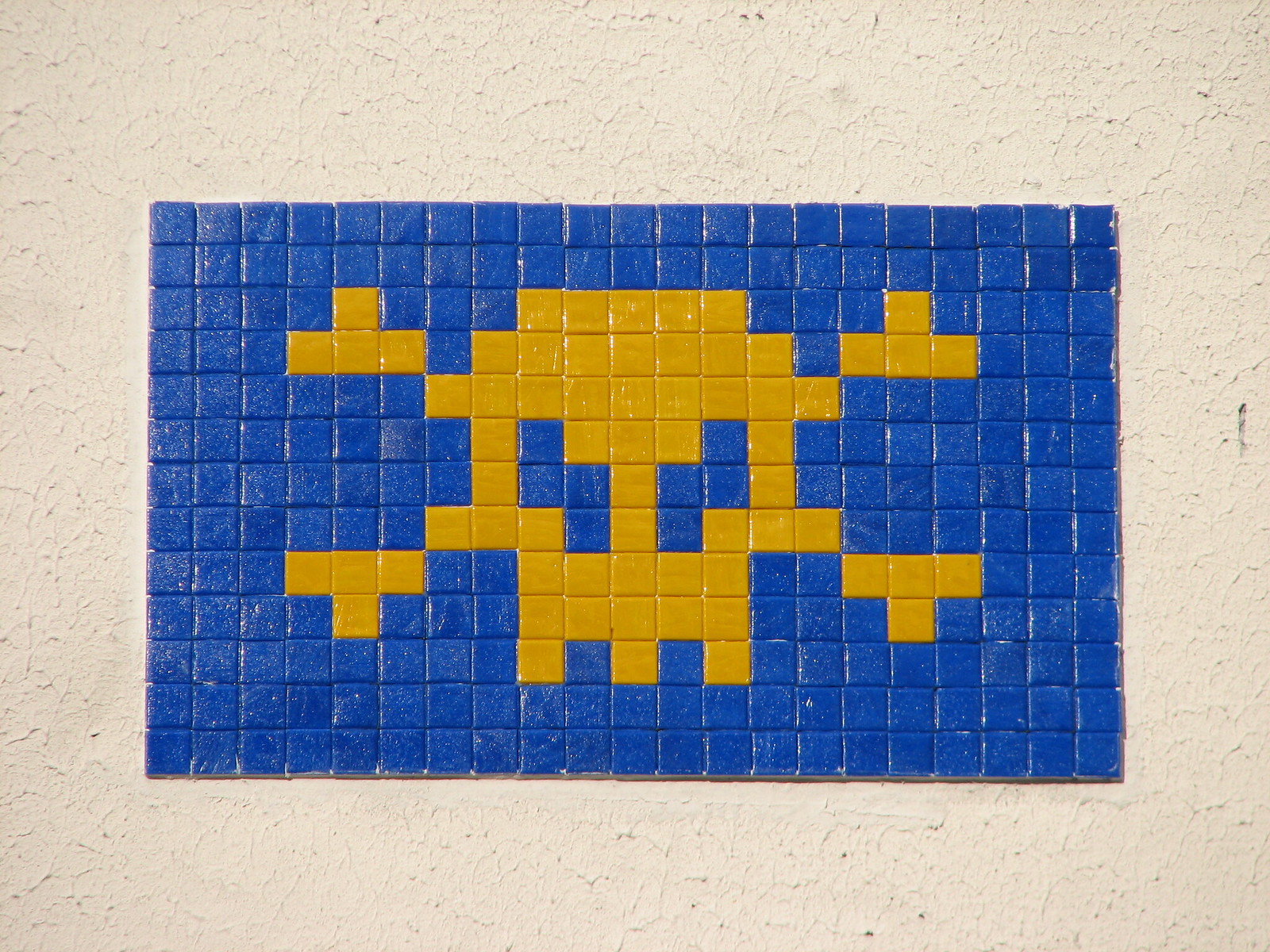The image showcases a tile mosaic mounted on a spackled ceiling. The mosaic is primarily composed of deep royal blue square tiles interspersed with golden yellow tiles, reminiscent of a vibrant school bus yellow. The intricate arrangement of the tiles forms a geometric figure that closely resembles a pixelated skull and crossbones. The skull is meticulously laid out with small teeth at the bottom, highlighted against the contrasting blue and yellow tiles, while the eye sockets are clearly defined in blue. The yellow tiles elegantly delineate the crossbones behind the skull, creating a striking and detailed visual effect.